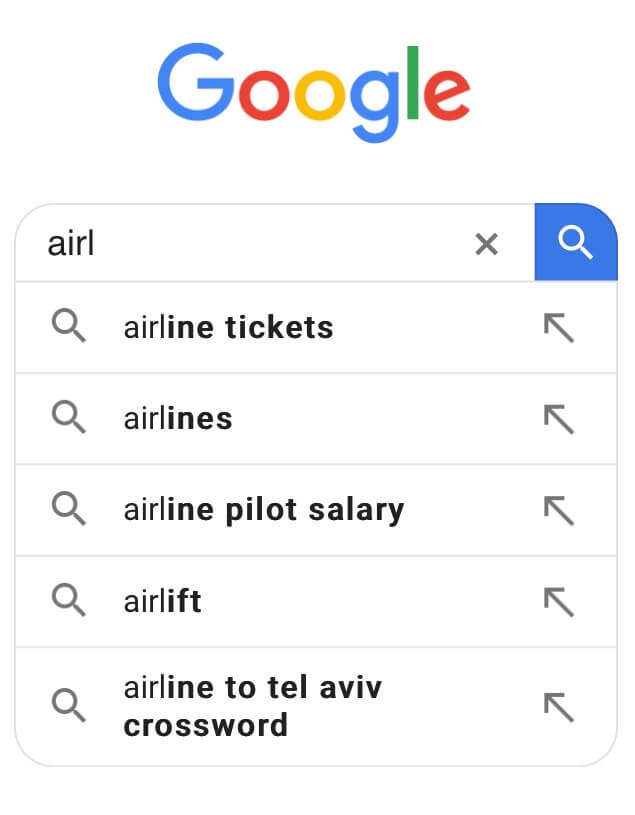The image displays a screenshot of a Google search page. The iconic Google logo is prominently positioned at the top center of the page. Below the logo is the search bar, where the user has typed "A-I-R-L." To the right of the search bar, there is an 'X' button designed to clear the entered text, followed by a magnifying glass icon, which serves as the search function button.

As the user types, Google suggests several autocomplete options. The top recommended search term is "airline tickets," followed by "airlines," "airline pilot salary," "airlift," and lastly, "airline to Tel Aviv crossword." Each suggested search term is accompanied by a small magnifying glass icon on the left side, indicating it is a search suggestion. On the right side of each suggestion, there is an arrow pointing up towards the top left corner, which allows the user to quickly select the suggestion and populate it into the search bar without immediately initiating the search.